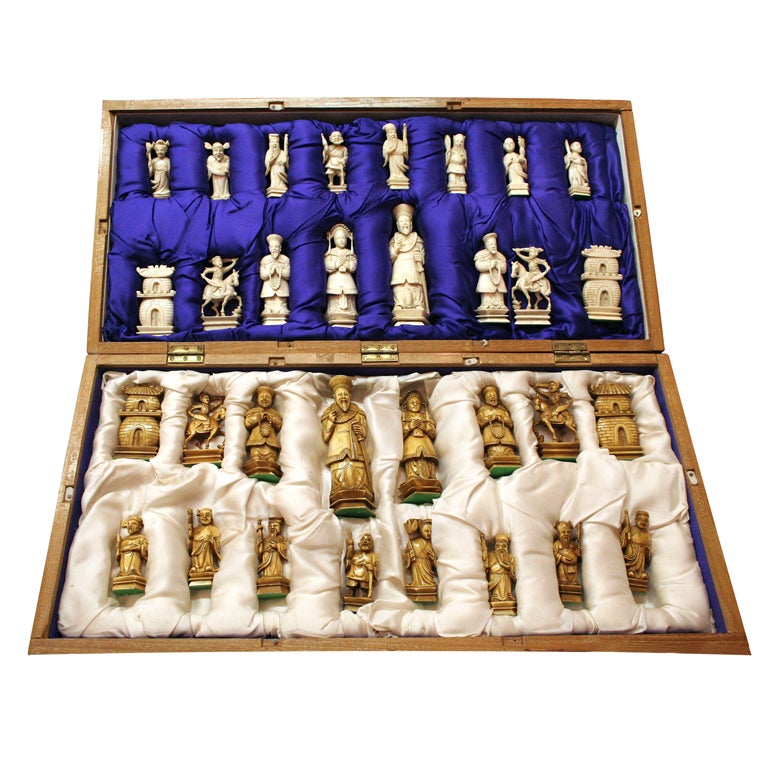The image depicts an opened, ornate wooden briefcase with three hinges. The case, which acts as a storage box for a detailed, old-fashioned chess set, is divided into two sections. The top half is lined with cushioned, silky blue fabric, while the bottom half features cushioned, silky white fabric. Each section is designed with individual slots to neatly hold the chess pieces. The chess pieces are exquisitely detailed and exhibit an Asian style, depicting emperors, buildings, and people on horses. The top half hosts white pieces, including the king, queen, rooks, bishops, knights, and pawns, while the bottom half holds a slightly yellow-tinted gold set. The colors of the pieces are reflective; although the yellow tint may be influenced by the fabric's hue, suggesting the possibility of them being crafted from ivory or a similar material. Overall, this set combines artistic craftsmanship with functional design, presenting an ancient, elegant chess set.